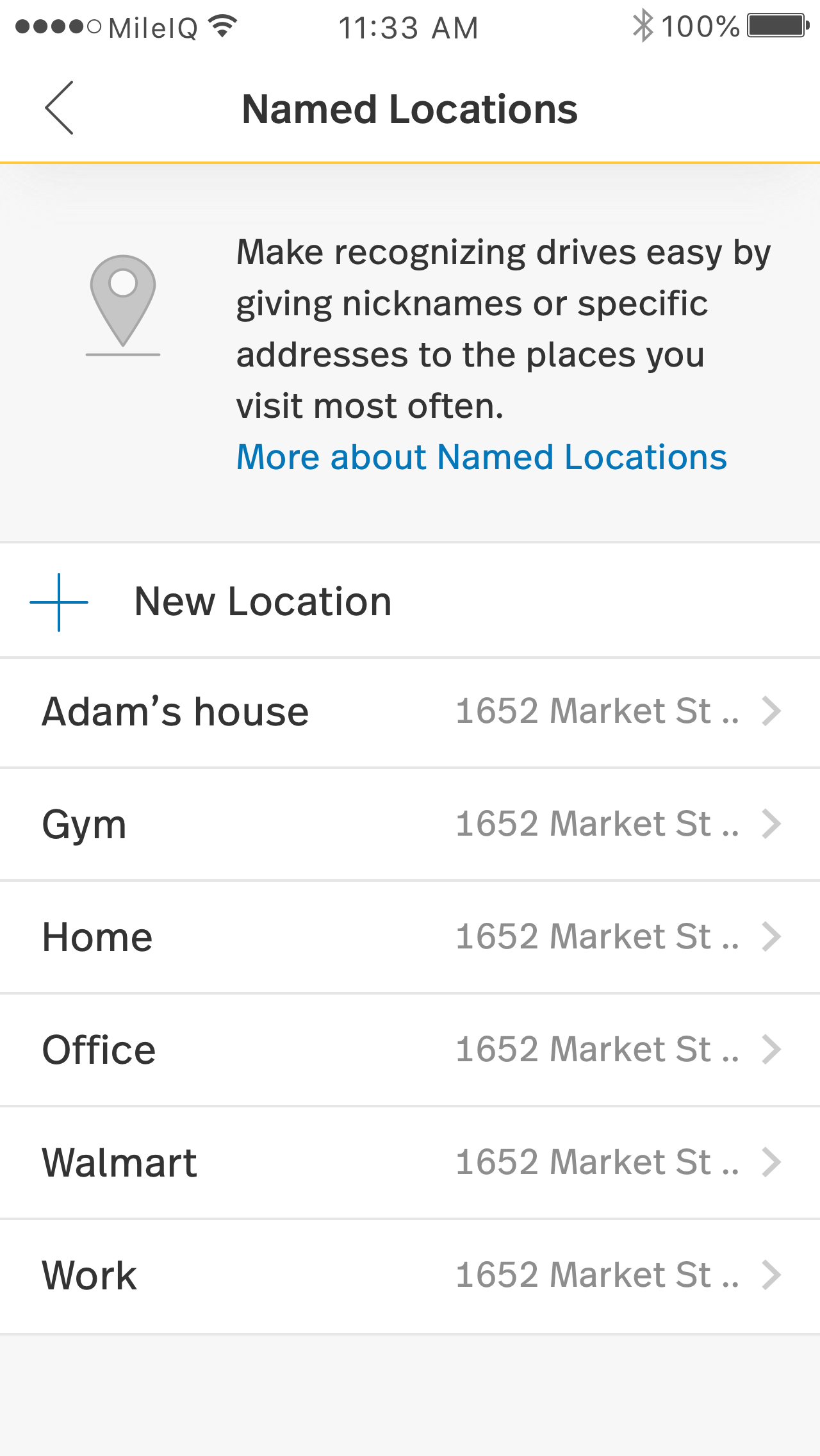This screenshot captures an iPhone display featuring various indicators of a highly functional and connected device. Positioned at the top left, the device boasts strong cellular reception with four out of five bars, serviced by MileIQ. The user is also connected to a reliable Wi-Fi network, with the time marked at 11:33 a.m. in the central top section. On the right-hand corner, Bluetooth is enabled, and the battery is fully charged at 100%.

The screen being viewed is organized under the section titled "Named Locations," prominently displayed in black font just below the time indicator. The overall background is predominantly white, accented by a light grayish-white box situated under the main title. To the left of "Named Locations," a back arrow icon hints at navigation options to a previous screen.

The descriptive text beneath the gray box encourages user interaction: "Make Recognizing Drives Easy by giving nicknames or specific addresses to the places you visit most often." Below this, a blue hyperlink labeled "More About Named Locations" invites users to learn more. The interface allows for the addition of new locations, showcasing already saved places such as "Adam's house," "gym," "home," "office," "Walmart," and "work." The structured and user-friendly layout ensures efficient management of frequently visited locations.